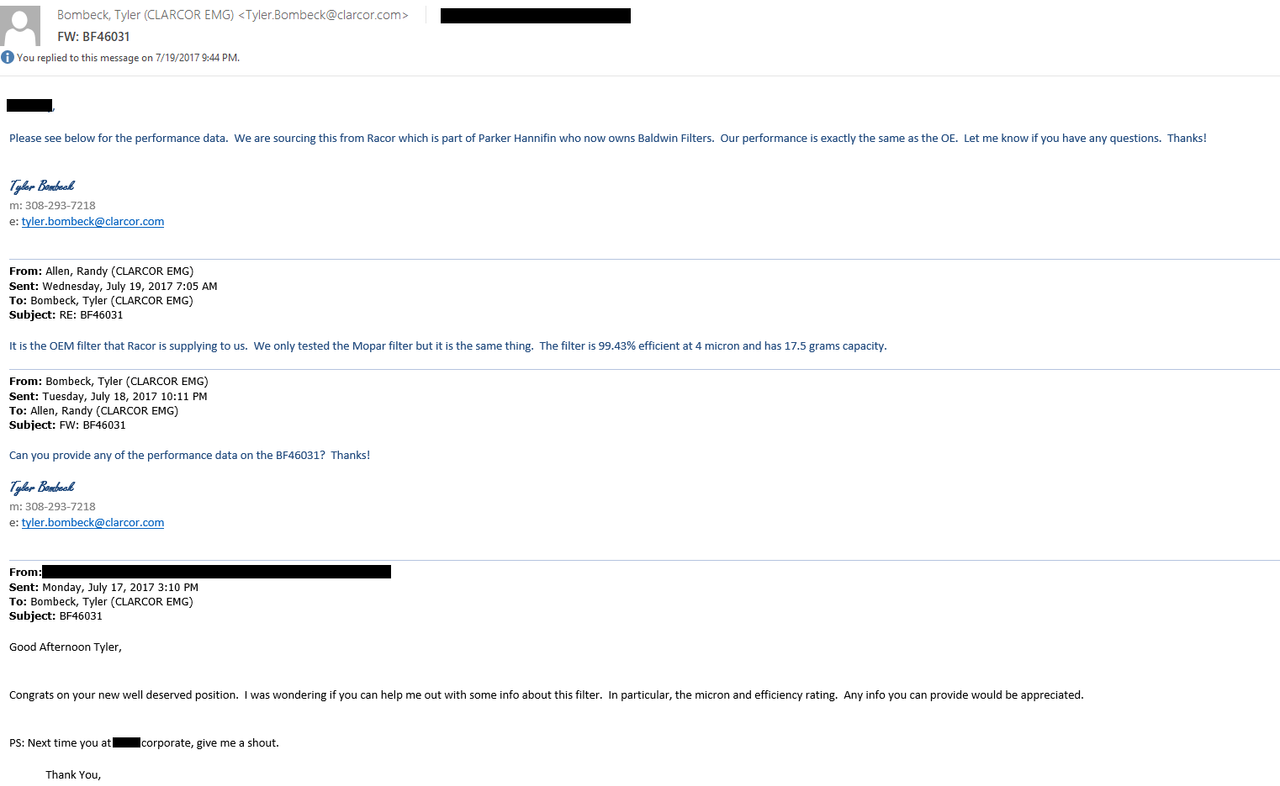The image depicts a screenshot of an email conversation. At the top, the sender's name, "Boomback Tyler," is visible, followed by a blacked-out section. The subject line reads "forward BF46031," indicating that the email has been forwarded. A timestamp is displayed, noting that the recipient replied to the message on July 19, 2017, at 9:44 PM.

Below the timestamp, another blacked-out section obscures some details. Further down, a formatted email header appears, containing fields labeled "From," "Sent," "To," and "Subject," followed by text that is partially obscured by a green line.

Subsequent email excerpts retain the same header format, with sections labeled "From," "Sent," "To," and "Subject," interspersed with gray lines. The final part of the email reveals more obscured content in the "From" field, with a message reading, "PS, next time you add [blacked out corporate], give me a shout, and thank you."